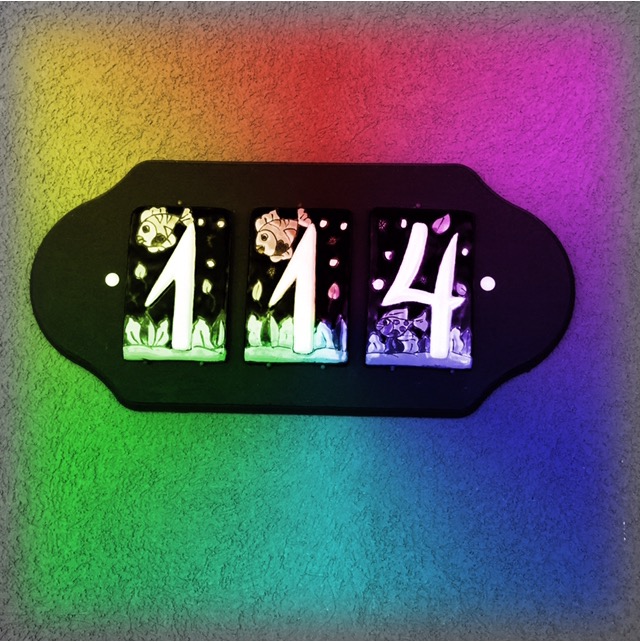This photograph captures a house address sign from an overhead perspective. The sign is black and rectangular with fully rounded ends. It is set against a white, rough 'gravel-like' background that’s visible at the extreme edges of the image. The surrounding wall features a vivid color gradient transitioning from yellow at the top left, to red and pink at the top right, then green at the bottom left, followed by cyan blue in the middle, and darker blue blending into purple towards the bottom right.

The central component of the image features the house address '114,' with each digit inlaid in separate rectangular sections resembling domino pieces. Each section depicts a vibrant scene from an aquarium with a fish and aquatic plants corresponding to each number. The first '1' is accompanied by a yellow fish with green plants, the second '1' showcases an orange fish with greenish-purple plants, and the '4' features a purple fish with purple plants. Illumination from an electronic device enhances the colors, casting a warm light on the yellow, orange, purple, and blue of the scene, adding an ethereal glow to the aquatic depictions.